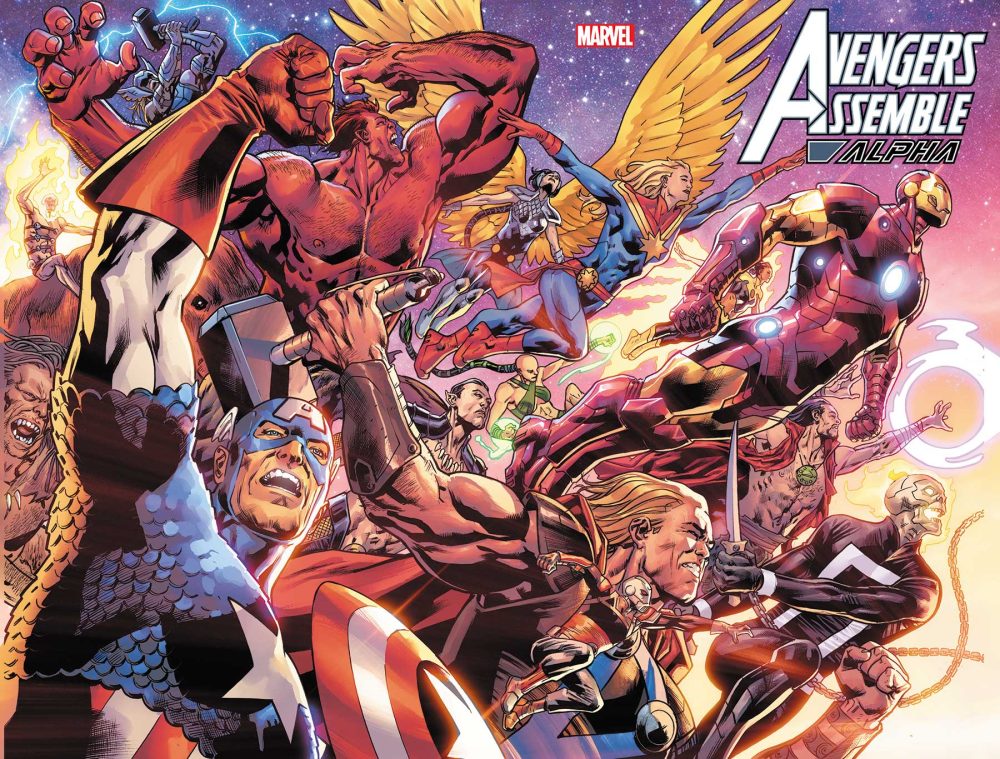This image is a detailed scan of what appears to be the cover of a Marvel comic, prominently showcasing the title "Avengers Assemble Alpha" in large white, all-caps text with a large 'A' and the word "Alpha" in black underneath, located at the top center. The artwork is densely packed with iconic Marvel superheroes climbing from the lower left to the upper right over a backdrop of a purple sky with starry and orange hues. 

In the lower left, Captain America stands out with his unmistakable blue suit, circular shield, and an 'A' emblazoned on his forehead as he raises his fist. Thor, with his signature long blonde hair and large hammer, is positioned right behind him. Beside them, Iron Man is depicted slightly beneath the title, possibly cradling or being engulfed by a blaze of fire, hinting at the presence of Ghost Rider. Other recognizable faces include Ant-Man, Red Hulk, and Namor, all rendered in dynamic poses. Their expressions and stances, from making fists to wielding weapons, convey an intense, action-filled scene. The heroes appear to be clustered together, emphasizing their assemblage for what might be an epic battle or pivotal event. Despite the intricate details, there is no additional text indicating the issue number, and the square format suggests it could be a cropped section of a larger image.